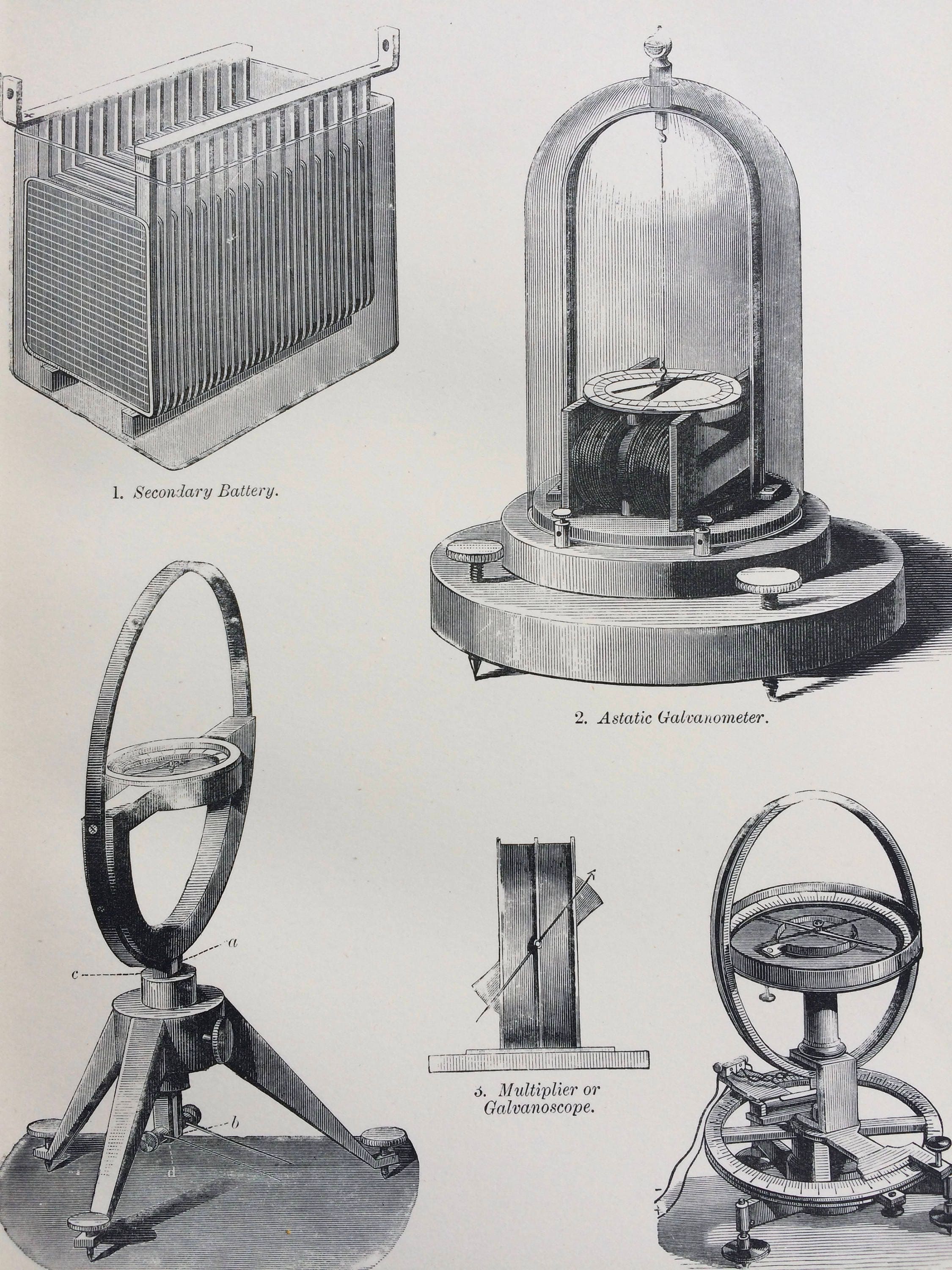This grayscale image, resembling a page from an old textbook, features detailed hand-drawn sketches of five vintage scientific devices, set against a light gray background. 

1. The first device, labeled "Secondary Battery," is positioned in the top left. It is a rectangular metal contraption with a mesh-like grid, similar to a radiator.
 
2. To the right, the second item, named "Astatic Galvanometer," appears as a dome-topped apparatus with a compass-like mechanism inside, resting on a wooden base adorned with screws and rivets.

3. In the center is a tripod-mounted device, featuring a hollow circular structure housing a meter that resembles a compass. This device is shown from a side view with an annotation indicating its rotational function and labeled as a "Multiplier or Galvanoscope."

4. The fourth item, unnamed, has a design akin to an intricate protractor mounted on a tripod with a domed circle above it, containing a meter parallel to the ground, suggesting use for precise measurement.

5. The fifth device, another unnamed tripod-based instrument, displays horizontal and vertical rings with a central compass-like instrument.

Detailed annotations and diagrammatic lines on these intricate sketches suggest their use in measuring or scientific applications, hinting at their historical significance in the realm of early scientific instrumentation.